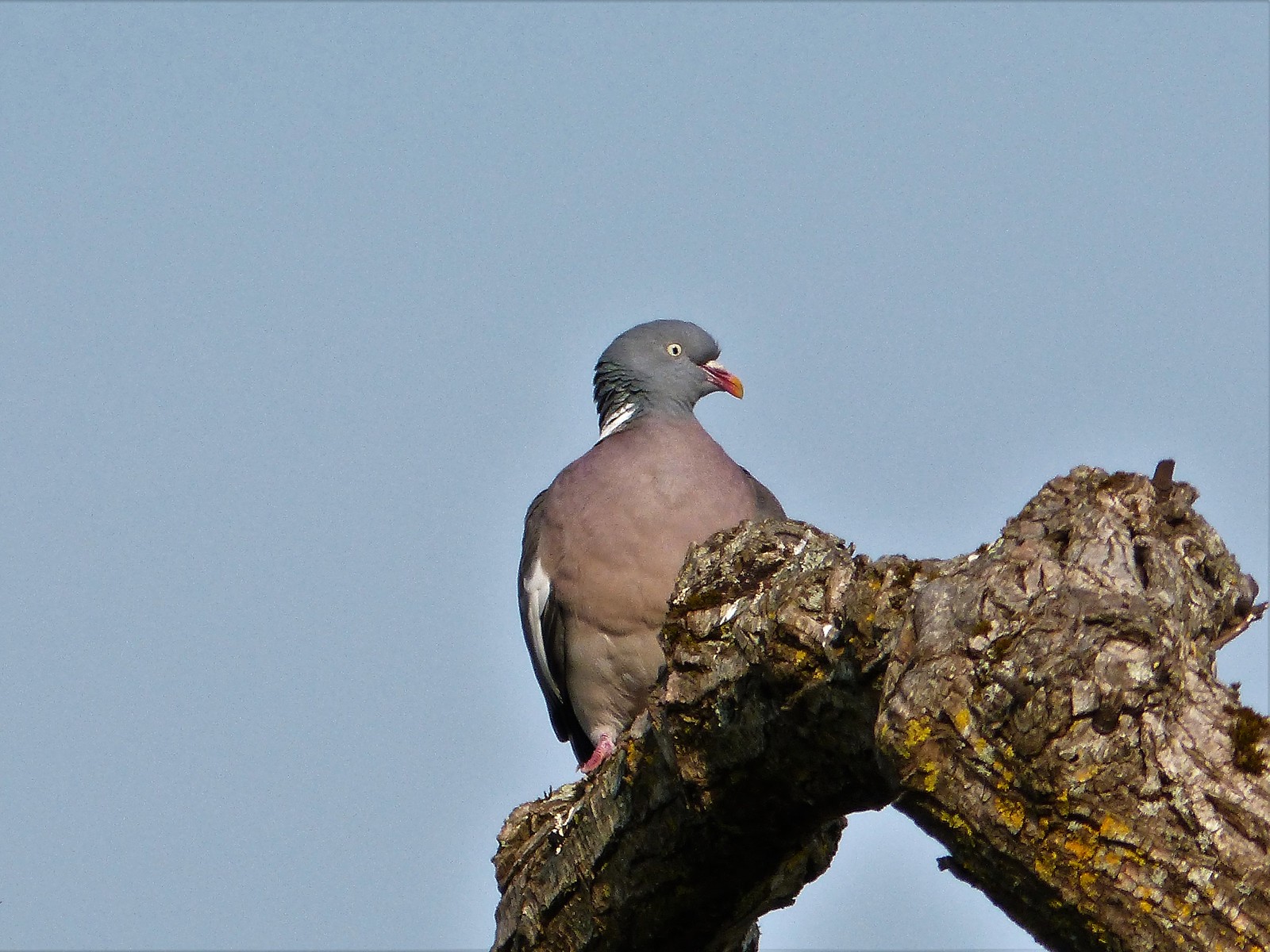This photograph captures a detailed close-up of a bird perched on a rugged, uneven tree branch, adorned with patches of moss and rust. The bird, with a slate gray head and a gradient body that transitions from light brown to a darker tan towards its bottom, features distinct physical characteristics such as a vibrant orange beak tinged with dark purple and a white ring around its eye. The bird's chest is light brown, showing some white under its wings and pink webbing on one of its feet. A side profile shot reveals the bird's body facing the viewer while its head turns to the right. The background showcases a dusty blue, clear sky, indicating that the photograph was taken during daylight hours, emphasizing the bird’s serene and restful pose.